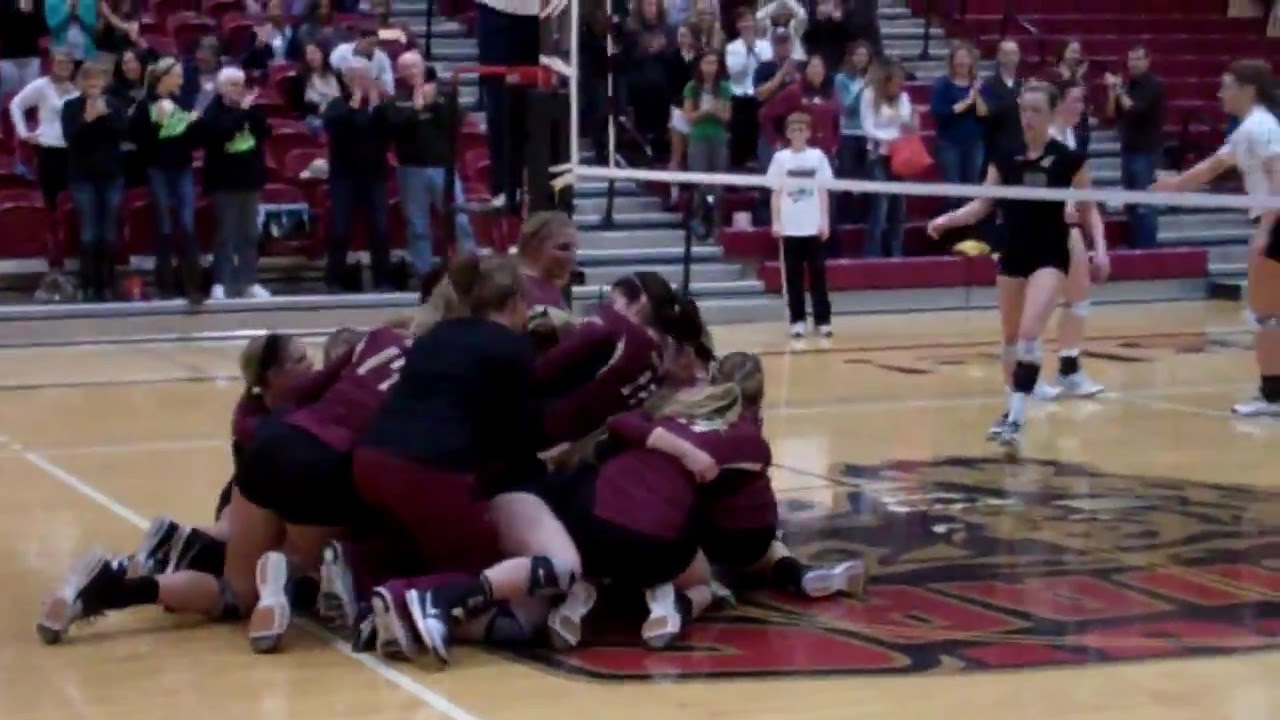The photograph captures an exhilarating moment during what appears to be a high school girls' volleyball game inside a gymnasium. At the center of the wooden gym floor, which features a visible yet indistinct red and gold logo, a jubilant team in maroon jerseys and black shorts is celebrating their victory by dogpiling on top of each other, smiles adorning their faces. To the right side of the volleyball net, a player from the opposing team stands in a black uniform, watching the celebration unfold through the white mesh. Most of the players have their hair tied back in ponytails accessorized with headbands, and they are all equipped with knee pads. In the background, metal stands are filled with spectators and a timekeeper—a young boy in a white t-shirt and black track pants—can be seen on the sidelines. There is also a coach in maroon pants and a black sweater observing the scene, highlighting an atmosphere filled with competitive spirit and communal support.